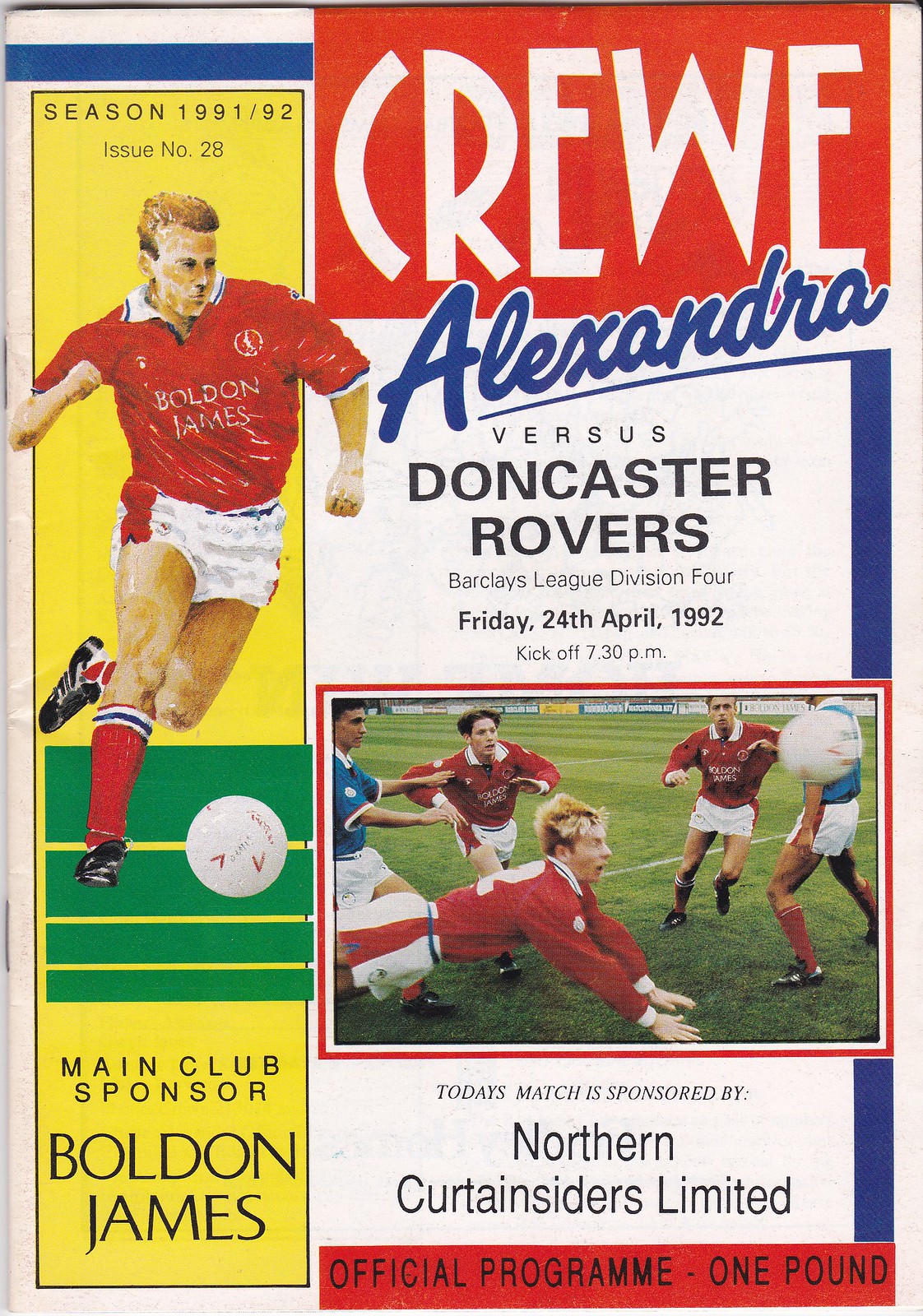This vibrant and detailed poster advertises a soccer match scheduled for Friday, April 24th, 1992, with a kickoff at 7:30 PM. Dominated by lively colors—reds, blues, whites, yellows, and greens—the left side features a footballer in old-fashioned style mid-stride against a yellow background. Sporting a red short-sleeved shirt, white shorts with a red stripe down the left side, and red socks with white and blue horizontal stripes at the top, he is shown about to kick a soccer ball on a green field. The player's reddish-brown hair and black shoes add further detail to his depiction.

Below the footballer, in bold black letters against the yellow background, the poster highlights the "Main Club Sponsor: Bolden James." 

Centered at the top on a red background in white font is "C-R-E-W-E," with "Alexandra" elegantly written beneath it in blue cursive. The text continues with "versus Doncaster Rovers," and adding "Barclay League Division IV" contextualizes the match.

An inset photo below shows teams in action, with players in red and white jerseys and a few in blue, leaping and diving for the ball. At the bottom, black letters on a white background announce, "Today's match sponsored by Northern Curtain Siders Limited," followed by "Official Program, one pound," against a red bar.